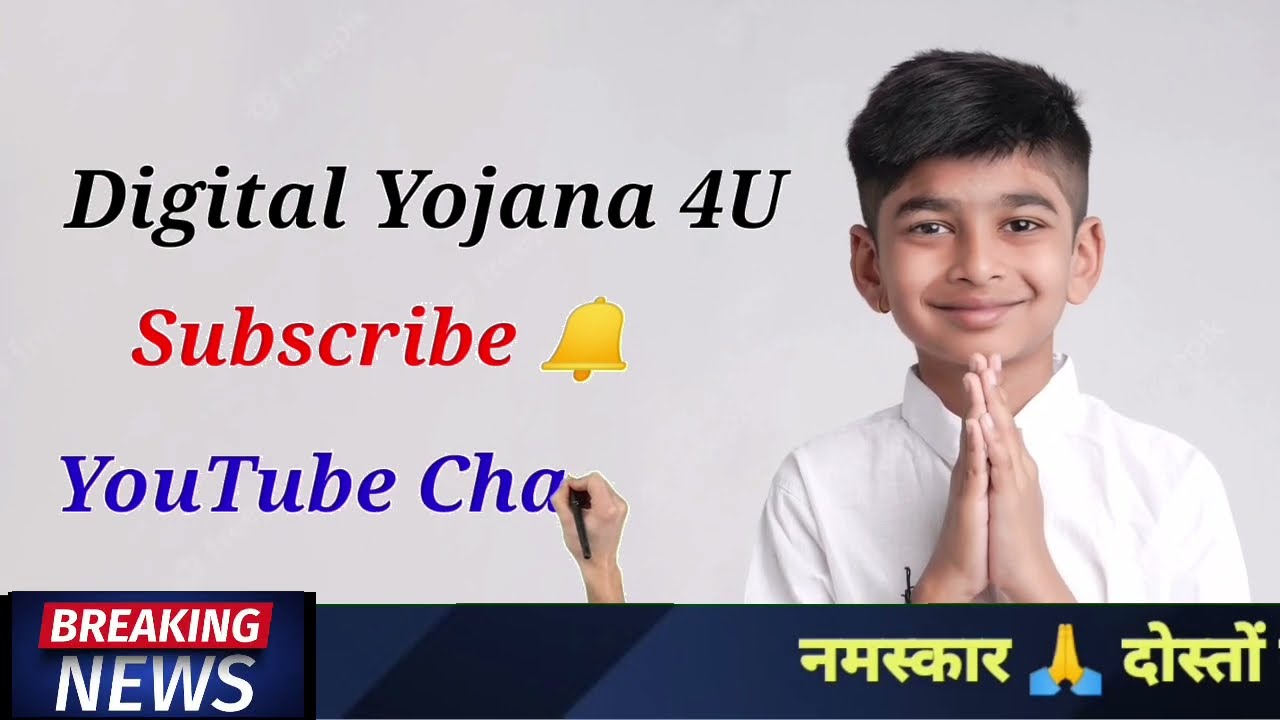The image depicts a young boy, likely between seven to nine years old, with dark brown hair and dark eyes, against a gray background. He is smiling, wearing a short-sleeved white dress shirt, and his hands are clasped together as if in prayer. Notably, his hair is parted on the left, shorter on the sides, and feathered to the side on the right.

The background and text elements clearly resemble a banner for a YouTube channel. On the left side of the image, italicized black lettering reads "Digital Yojana for you." Below this, in italicized red text, the word "subscribe" is displayed next to a yellow bell icon. Further down, dark blue text spells out "YouTube CHA," with a hand holding a pen appearing to continue writing.

At the bottom of the image, a blue banner with a black border contains the text “Breaking News.” “Breaking” is in white, all-capital letters within a red box, while “news” is in white. On the right side of the banner, there’s an icon featuring praying hands with blue sleeves and yellow hands, accompanied by text in an unidentified language written in yellow. The collective elements suggest a professional, perhaps promotional, design setup for a YouTube channel involving news updates and calls to subscribe.